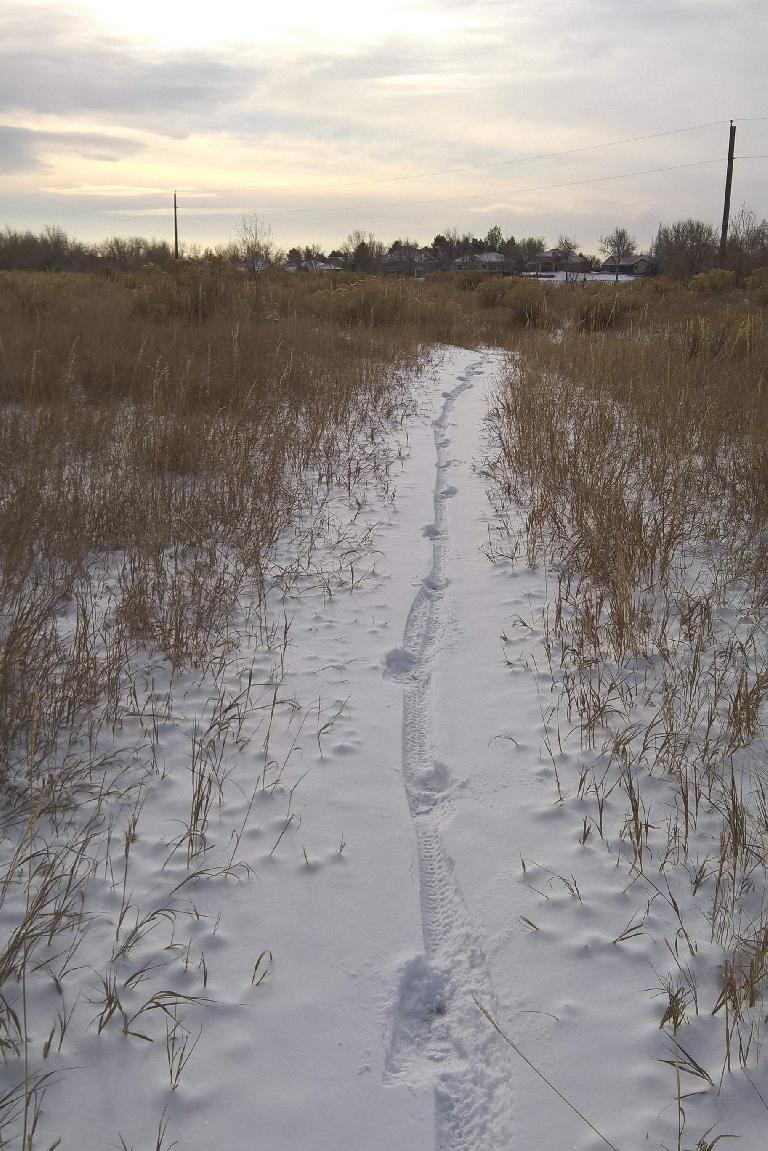The image is a vertically aligned rectangular picture taken in an outdoor field, possibly a park. The scene is dominated by tall, dead brown grass or weeds, densely covering both sides of a snow-covered trail. This trail, positioned centrally and starting from the bottom, stretches upwards past the middle of the image. The trail shows signs of varied use, evidenced by narrow wheel tracks and a few footprints, potentially indicating that it has been traversed by a bicycle.

In the background, just beyond the field, a white structure, possibly a house, can be seen. The composition also features several power lines and poles, crossing horizontally from left to right. The sky above is mostly cloudy, blending shades of pink, gray, and white. The image palette includes the earthy tones of the dead grass and subtle hues in the cloud-filled sky. There's no text on the image, focusing purely on the natural and man-made elements within this tranquil, wintery landscape.